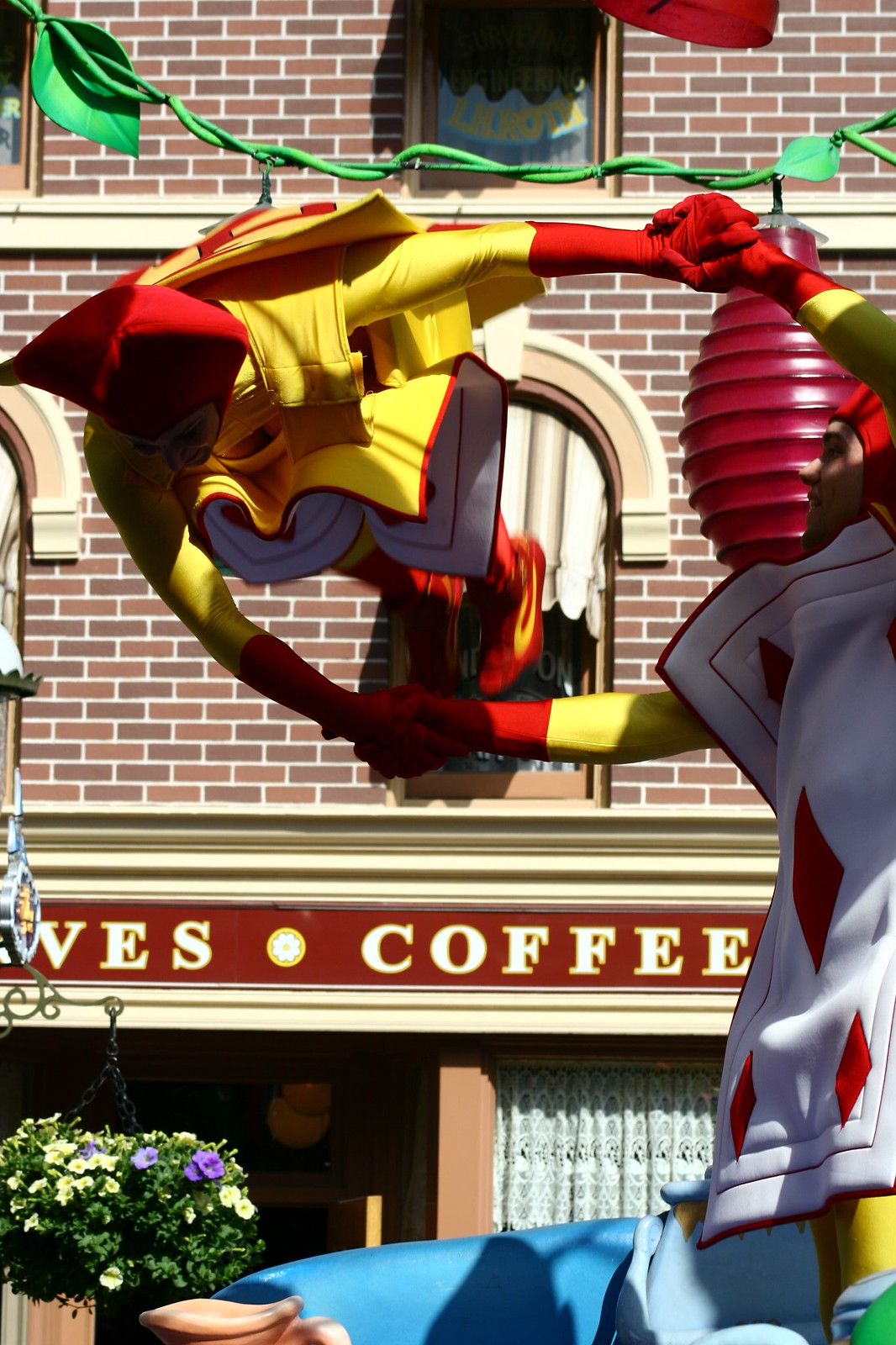A red and yellow device, possibly a mascot or promotional object, extends from the top of a brick coffee shop building. The building, adorned with window arches, features a sign with the word "Coffee" prominently displayed. At the bottom left of the scene, several potted plants add a touch of greenery. A green ribbon stretches across the top, seemingly attached to a mysterious red ball. The overall structure and elements suggest a quaint, welcoming atmosphere despite the unclear function of the suspended object.